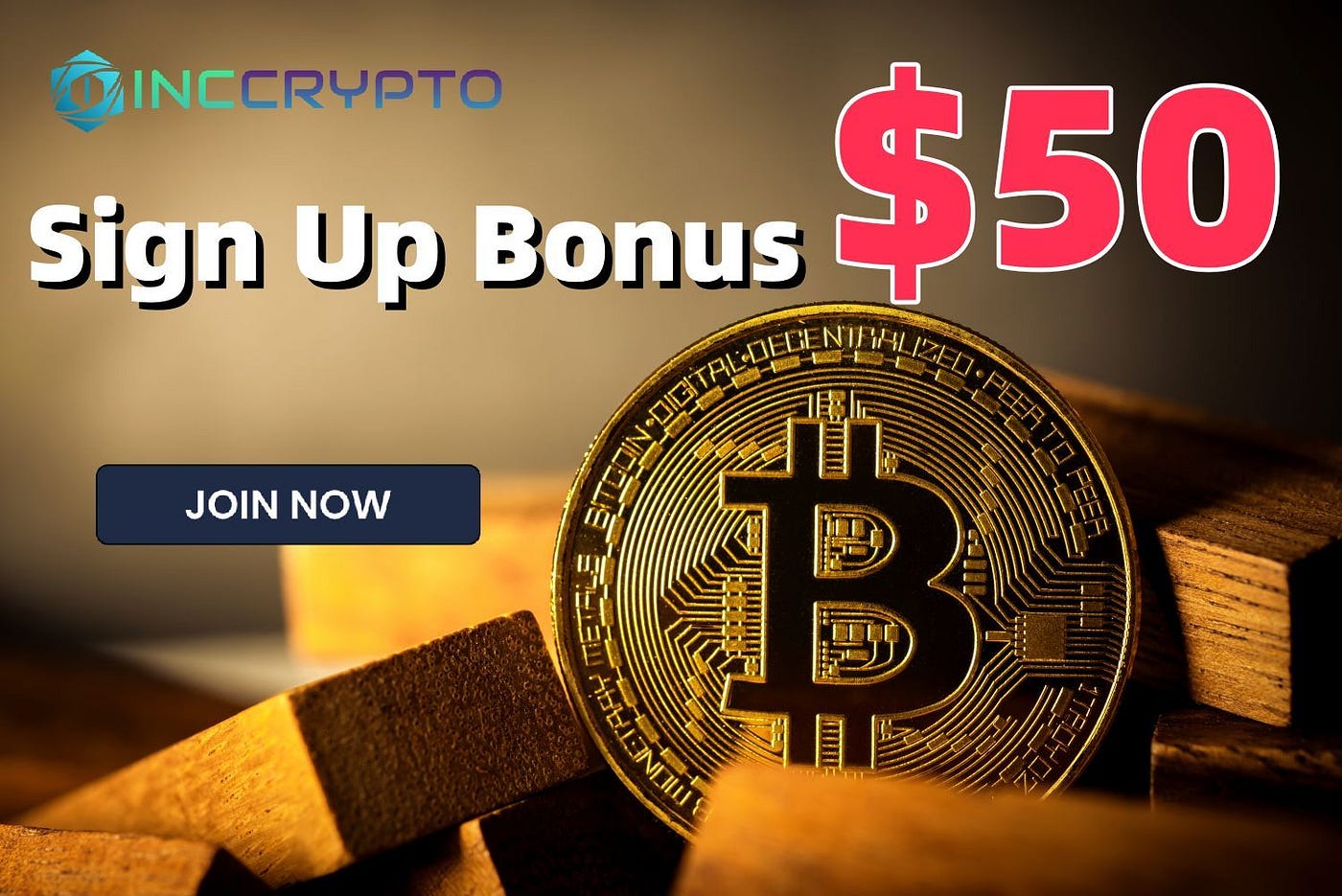The promotional banner for cryptocurrency is a neat and clearly designed rectangular advertisement, with the top and bottom sides twice as long as the left and right. At the top left corner, the banner features text that reads "INC" in green, followed by "crypto" in blue, accented by a teal emblem and a blue hexagonal shape. The upper right corner displays "$50" in bold red text with a white border. Below the "INC crypto" text, in white font with a black outline, the words "sign up bonus" are prominently visible. Central-left in the banner is a blue rectangle featuring the call-to-action "join now" in white text. 

Dominating the visual center of the image is a physical representation of Bitcoin—a large gold coin with a prominent "B" in the center, traversed by two parallel lines similar to a dollar sign, and surrounded by intricate circuit patterns. Around the edge, the coin reads "Bitcoin Digital decentralized peer-to-peer." The coin is nestled within a large pile of small wooden rectangular blocks. Overall, the banner communicates an enticing $50 sign-up bonus for new users, designed to attract attention even in competitive advertising spaces like social media feeds.